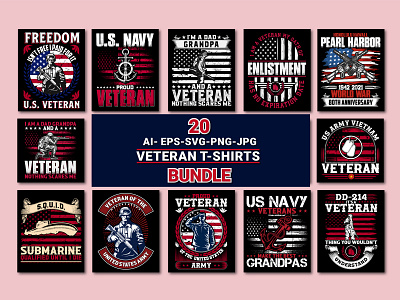This image is a square mock-up showcasing a collection of 20 veteran-themed t-shirt designs, prominently displayed on a pinkish background. The central area features a horizontally rectangular blue box that reads, "20 AI, EPS, SVG, PNG, JPG, Veteran T-Shirts Bundle." Surrounding this central text are numerous t-shirt designs primarily in red, white, and blue—colors symbolizing patriotism. The designs include diverse themes such as "Freedom," "U.S. Veterans," "U.S. Navy Veteran," "Grandpa and a Veteran," "Enlistment," "Pearl Harbor," "U.S. Army Vietnam Veteran," and "U.S. Navy Grandpas." Various images like soldiers, submarines, and battle tags enhance the patriotic and military focus of the collection, clearly targeted at veterans and their families.